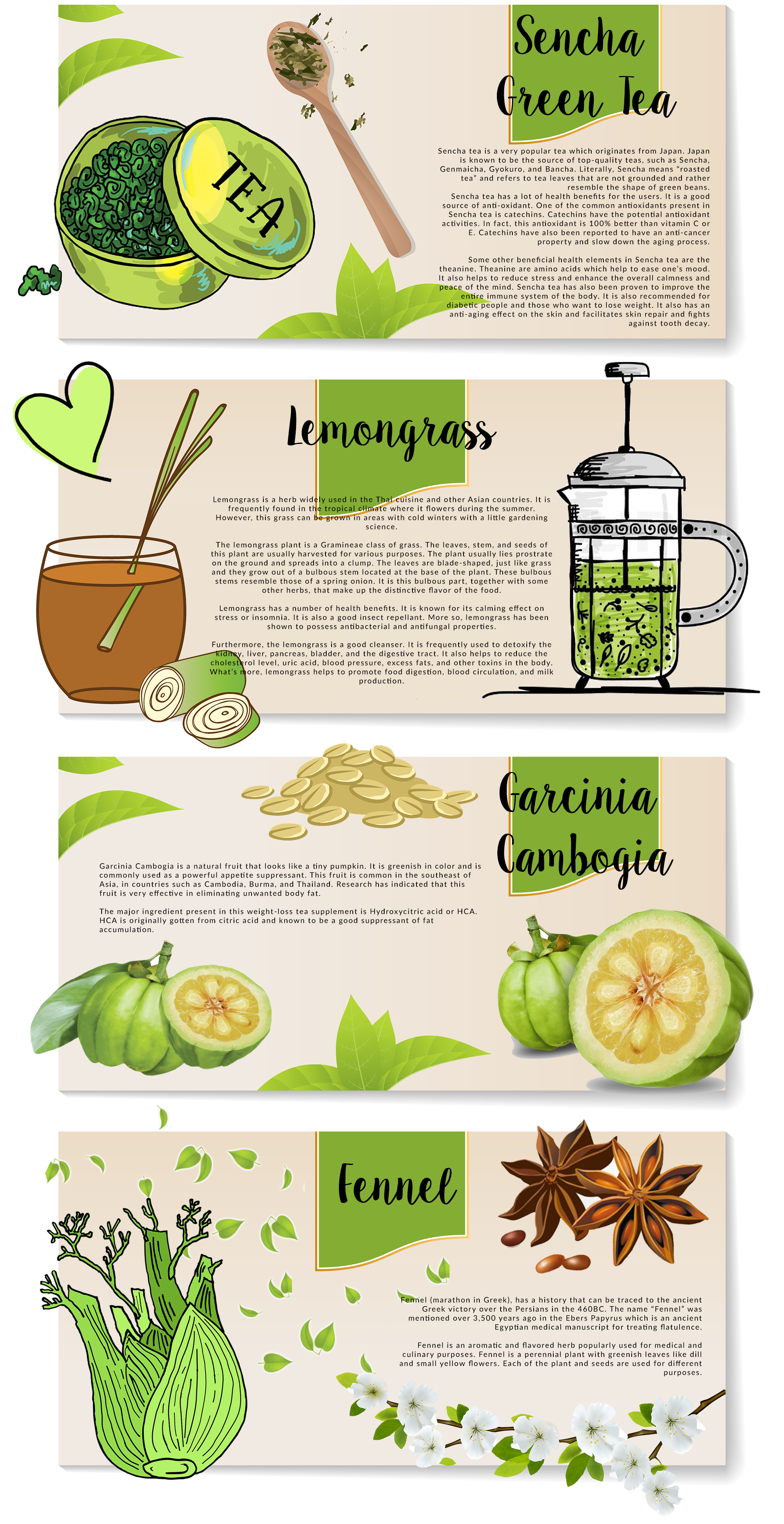This image appears to be a detailed illustration from a magazine or brochure page, featuring various green herbs and edible plants, each accompanied by informative descriptions and stylized, cartoonish yet realistic drawings. At the top, there is a depiction of Sencha green tea, which is a popular tea originating from Japan. The accompanying text highlights its health benefits, stating that it is rich in antioxidants such as catechins, which are more potent than vitamins C and E and possess anti-cancer properties as well as the ability to slow the aging process.

Below that, there is an illustration of lemongrass, along with instructions and imagery showing how to prepare lemongrass tea. This section includes a picture of a blender, a heart symbol indicating its health benefits, and a cup with lemongrass stalks.

Next, the image covers Garcinia cambogia, depicting the green and yellow fruit alongside a description of its uses. Though limited details are provided, it suggests that this plant is used for some form of tea or culinary preparation.

At the bottom, there is an illustration of fennel, showing a large bulb with green leaves. The fennel section likely includes information on how to use the plant, potentially in tea, though specific instructions are not detailed here.

Overall, the page combines artistic drawings with practical information on the benefits and preparation of each herb and plant, creating an engaging and educational layout.